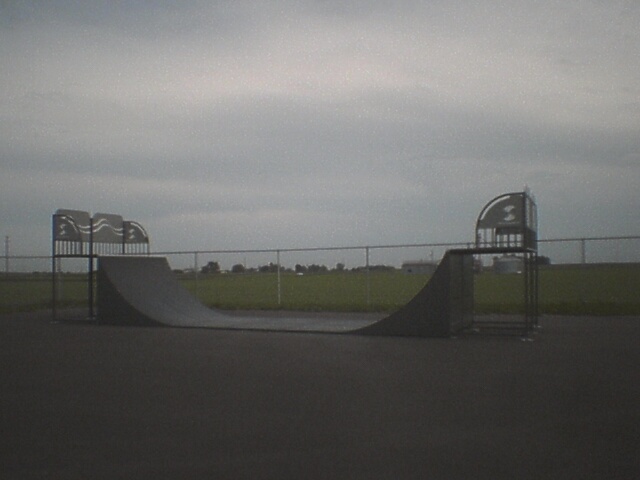The image depicts a skate park captured during an overcast evening, lending a dim, dusky atmosphere to the scene. Central to the picture is a prominent gray double-sided vert ramp, made of wood with metal-framed platforms on either side for skaters to rest or jump from. The ramp is situated on a flat, asphalt-paved area, enclosed by a chain-link fence that delineates the skate park's boundary. In the background, beyond the fence, an open grassy field stretches out, leading up to a line of trees and a few distant buildings on the right side. The sky is filled with gray, heavy clouds, contributing to the overall dark and subdued lighting of the scene. The park appears empty, with no people visible, emphasizing the quiet, almost solitary ambiance of the evening.